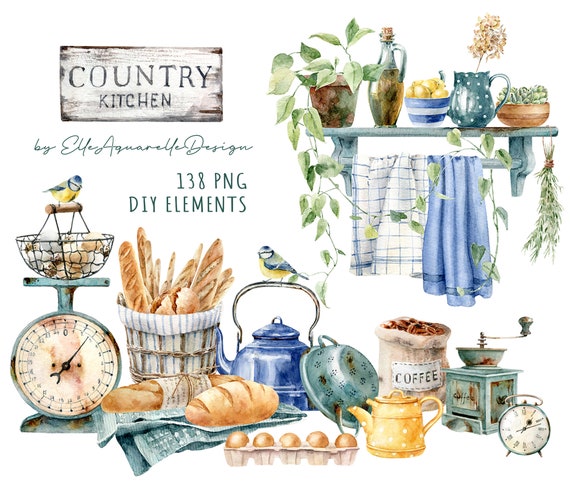This detailed color illustration by L. Annabelle Design titled "Country Kitchen" features 138 PNG do-it-yourself elements. Dominating the upper left corner, a sign reads "Country Kitchen by L. Aquanel Design." To the far right, a charming shelf showcases various rustic items: a creeping vine from a potted plant, a jug of olive oil, a blue and white bowl of pears, a green polka-dotted pitcher with a plant, and a small brown bowl housing a succulent. Below the shelf hangs a rod with blue and white dish towels and a sprig of an unknown herb or plant.

In the forefront, an antique scale holds a basket of eggs, with a small yellow and blue bird perched on its handle. Nearby, a wicker basket filled with baguettes partly covered by a white and blue towel rests alongside extra baguettes. A blue tea kettle is adorned with another small blue and yellow bird. The scene also includes a leaning colander and five eggs arranged meticulously in the foreground. Complementing the country theme are additional items such as a yellow polka-dotted tea kettle, an open bag of coffee beans, an old-fashioned coffee grinder, and an alarm clock set to 1:11, AM or PM unknown. This illustration evokes the cozy and nostalgic charm of a mid-20th-century country kitchen, filled with decorative yet functional pieces.